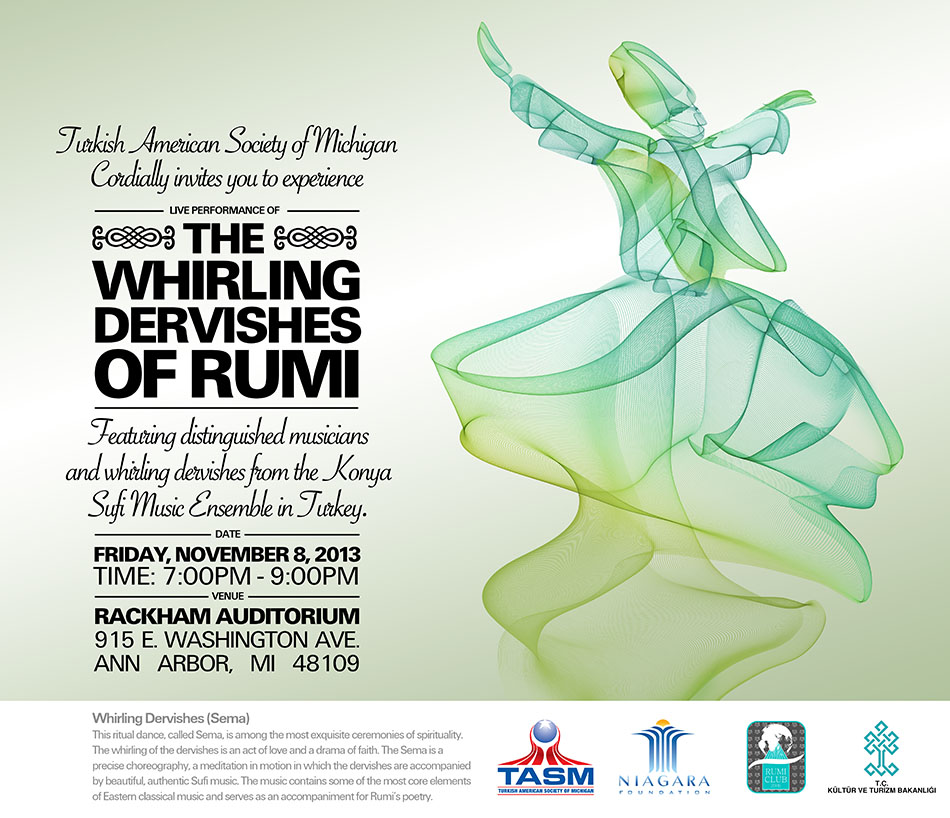This advertisement poster, featuring a light cream background, promotes a live performance by the Whirling Dervishes of Rumi, organized by the Turkish American Society of Michigan. The left column contains event details in a mix of black cursive, bold, and all-caps fonts, detailing the date, Friday, November 8, 2013, and the time, 7 p.m. to 9 p.m., at Rackham Auditorium, 915 East Washington Avenue, Ann Arbor, Michigan 48109. The text invites guests to experience distinguished musicians and whirling dervishes from the Konya Sufi Music Ensemble in Turkey. The right column showcases a whimsical and abstract geometric vector art depicting a man in a tall hat twirling, rendered in various shades of green and yellow, some parts transparent, portraying the dancer's fluid motion. The figure faces right and appears to be looking upwards with hands spread. At the bottom, a white horizontal band contains small text disclaimers and sponsor logos. The overall design blends color illustration with graphic design on a gradient light green to white background.